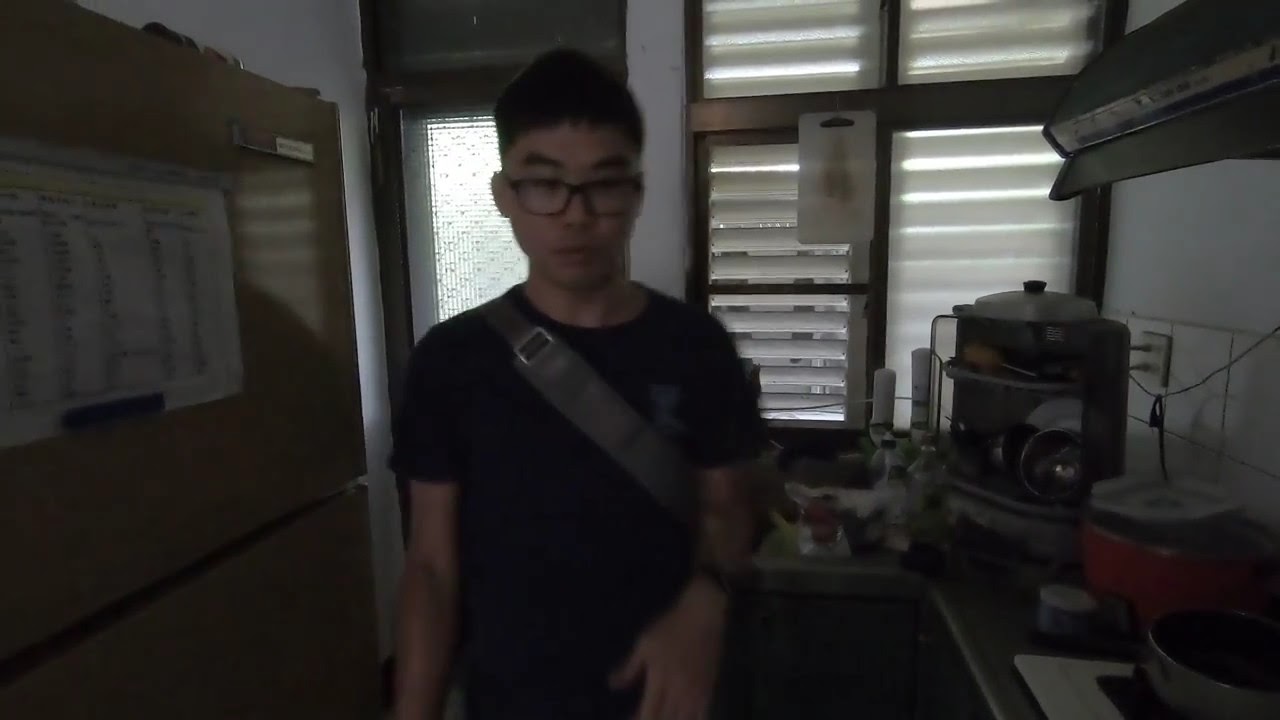In this dimly lit small kitchen, a young Asian man stands in the immediate foreground. He is wearing square black-rimmed glasses, a black t-shirt, and a book bag with a green strap draped over his left shoulder. His spiky black hair adds a touch of style as he poses for a selfie, his right arm slightly raised while his left arm rests by his side. To the left of the man, a refrigerator-freezer combo with a chart attached to the freezer door can be seen. On the right, a stovetop with a pot on one of the burners and a crock pot sits on the countertop. The countertop extends below a window with closed blinds. In the corner by the window, a coffee machine and other small kitchen utensils are visible. Additionally, a white door with metal bars in the window area is partially obscured by the man. His casual stance and the kitchen setup suggest a cozy, lived-in apartment space.